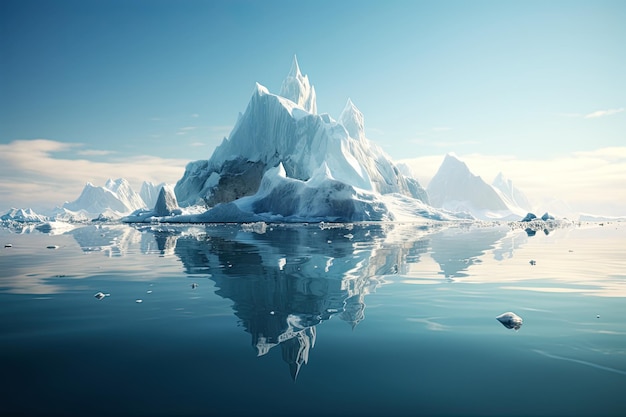The artwork presents a stunning and highly realistic depiction of an Arctic or Antarctic landscape. Dominating the scene is a colossal ice mountain, its pure white and strikingly pristine peak contrasting sharply with the dark gray and blue hues near its base, perhaps indicating rocky outcrops. At its foot lies a body of serene, crystal-clear blue water that flawlessly mirrors the surroundings, including the majestic mountain and pieces of floating ice. 

To the sides of the central mountain, additional peaks emerge; one on the right intriguingly resembles a pyramid with shades of gray and light blue, while another sits further in the distance. The sky overhead is a perfect expanse of clear blue, punctuated by a few wisps of white clouds near the horizon. This daytime scene, characterized by its vivid colors and intricate details, not only captures the chilly beauty of a polar environment but also suggests the allure of such a location as a piece of wall art, suitable for a rectangular frame. The overall composition, with its calm waters and majestic ice formations under a bright sky, conveys a profound sense of tranquility and natural grandeur.